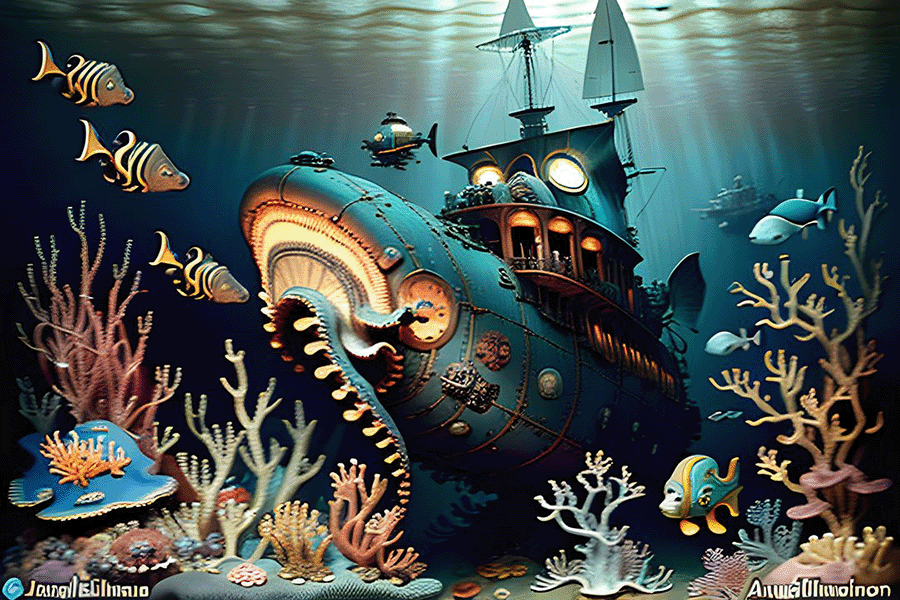This is an intricately detailed computer-generated image, possibly AI-rendered, featuring a fantastical, steampunk-style submarine submerged in an underwater seascape. The submarine, adorned with sails and masts, has a dark blue and teal color scheme with yellow accents. It boasts multiple levels, portholes, and even a porch. Metallic rivets and seams accentuate its mechanical appearance. A notable feature is an octopus tentacle protruding from the front, seemingly investigating the vessel.

The underwater scene is vibrant and teeming with marine life. On the left side, three yellow and black striped fish swim amid a colorful array of coral in shades of pink, yellow, and peach. On the right side, a blue and yellow fish, appearing almost three-eyed, flits around sparser coral that dominantly displays hues of yellow and blue. The seabed is covered with an assortment of bright, colorful crustaceans and corals. In the background, additional, smaller submarine vessels can be seen, enhancing the depth of this fantastical seascape.